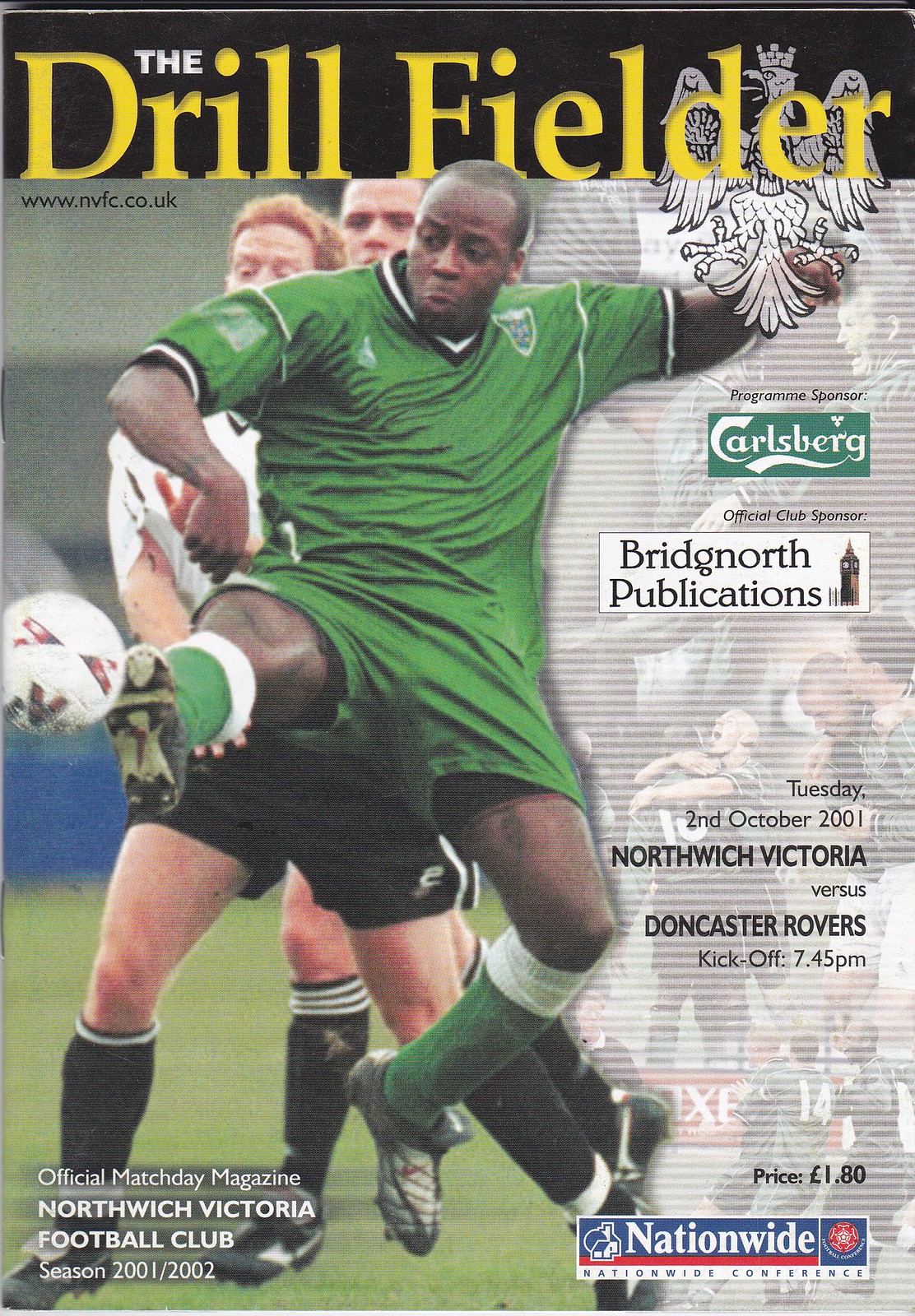The cover of the magazine, "The Drill Fielder," prominently features a bold, gold title against a black background at the top. "The" is written in small, white capital letters just above the "R" in "Drill Fielder." To the right, a line art eagle is subtly integrated beneath the word "fielder." Below this is the URL www.nvfc.co.uk in fine print. The central part of the cover exhibits an action-packed photograph of a soccer match. Dominating the foreground is an African player clad in a dark green jersey, green shorts, green socks, and black shoes, captured mid-kick with a red and white ball. Behind him, two white male players in black shorts, black socks, and white t-shirts are visible. Along the right margin, sponsor information is displayed with a striped gray and white background. Logos for "Carlsberg" (inside a green rectangle indicating a program sponsor) and "Bridge North Publications" (inside a white rectangle as the official club sponsor) are noticeable. The date "Tuesday, 2nd October 2001," the event "Northwich Victoria vs. Doncaster Rovers," and the kickoff time "7.45 PM" are prominently listed in the design. At the bottom of the cover, a blue rectangle with the word "Nationwide" in white lettering capped with a red underline denotes the Nationwide Conference.